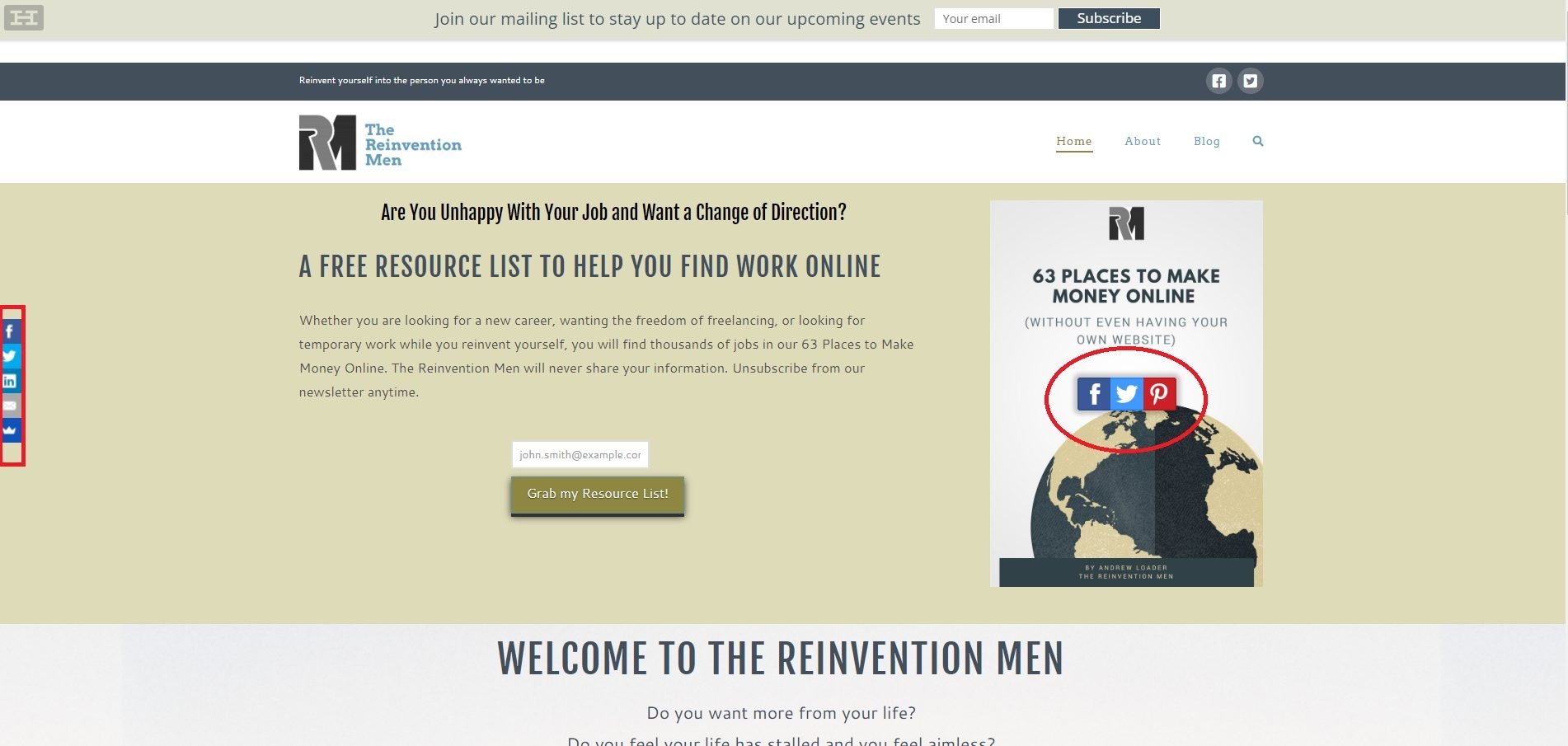This is a screenshot of a website, although the small size makes it difficult to discern details without zooming in. In the top left corner, there is the website's logo, comprised of the cleverly interwoven letters "R" and "M" from the name "Reinvention Men." The "R" integrates seamlessly into the start of the "M," creating an elegant and creative design.

The main background of the website is predominantly white, while the top banner is a soft greenish-cream color. The text on the banner is a mixture of light and dark green hues, stating, "Join our mailing list to stay up to date on our upcoming events." To the top right of this banner, a field is provided for users to input their email address, accompanied by a green "Subscribe" button.

Below this, there's a dark green banner featuring bold white text that reads, "Reinvent yourself into the person you always wanted to be." To the right of this, there are icons linking to Facebook and Twitter.

The navigation menu below this dark green banner includes tabs for "Home," "About," and "Blog." The "Home" tab is currently highlighted in the same greenish-cream color as the top banner, indicating its active status.

In the middle section, prominent text asks, "Are you unhappy with your job and want to change your direction?" Below this question, the website offers "a free resource list to help you find work online," followed by additional descriptive text outlining their mission and services.